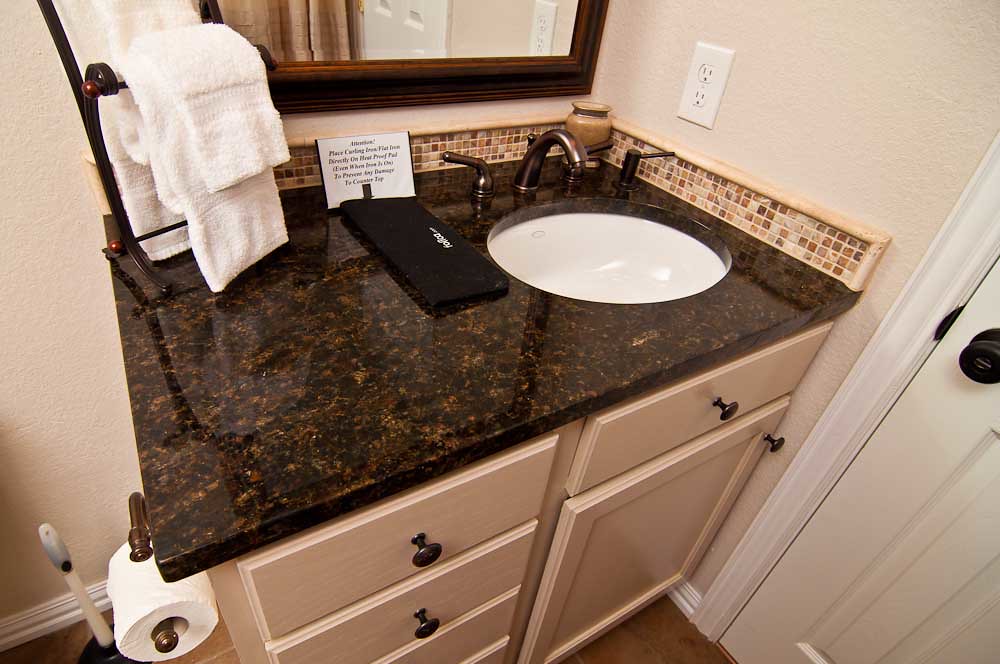The image depicts a bathroom sink area, possibly located in a hotel due to its compact and utilitarian setup. The photograph is taken from an overhead perspective that captures both the sink and the lower portion of a closed door to the right side of the frame. The door features a dark-colored doorknob and latch.

Underneath the sink, there are tan-colored drawers and cabinets, providing storage space. The sink countertop is designed in a brown and gold Formica surface, adding a touch of elegance to the setting. The sink bowl itself is circular and pristine white, contrasting with the brass-colored metal handles and faucet.

To the left of the sink, a hand towel holder supports a couple of neatly folded white towels. Behind the sink, in the top left corner, a sign with black lettering on a white background is visible, although the text is unreadable. Beside the sign, a small black rectangular object, likely a shaving kit, is placed.

A mirror mounted above the sink reflects parts of the bathroom, showing a tan shower curtain on the left and a white object on the right. Additionally, a vase decorates the corner of the sink, adding a decorative element. An American-style electrical outlet can be seen to the right of the sink, providing convenient access to power.